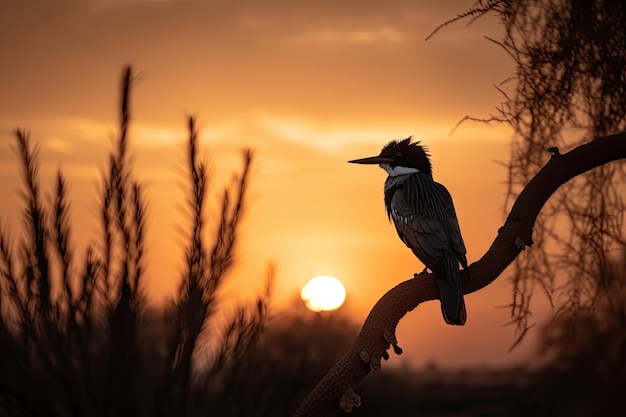This photograph captures the soft, warm hues of a sunset, with the sky awash in shades of orange and subtly blending into golden pink closer to the sun, which rests low on the horizon, casting a delicate, dim glow. The contrasting silhouettes of plants frame the scene: wispy, elongated branches shoot upwards on the left, while undefined, dangling vines drape from the upper right. Dominating the composition is a curvaceous branch that spans from the bottom center to the upper right, upon which perches a regal kingfisher. The bird, depicted in profile facing left, features a striking appearance with its long, pointed beak, dark plumage, and distinctive spiky head feathers. The kingfisher's white lower jaw and neck contrast sharply with its dark body, while its square tail feathers complete its elegant silhouette against the dimming sky.